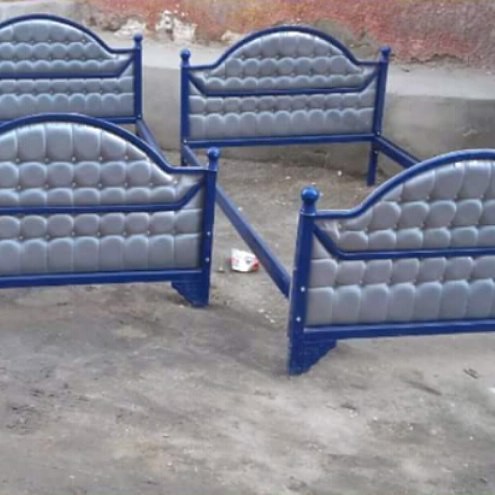A photograph captures two identical, empty bed frames placed outdoors on a dirty, partially concrete, and debris-laden ground. These bed frames are designed with a vibrant blue metal structure, featuring both headboards and footboards padded with a gray, plush-like cushioning. The frames lack mattresses or box springs, revealing the bare blue metal slats. Each frame has rounded knobs at the top, and the legs are angled into a triangular shape. The scene appears to be in an industrial or neglected area, indicated by the dirty surroundings and litter, including a distinct white and red piece of trash beneath one of the frames. In the background, there's a weathered wall with a rusted, reddish-brown hue, exposing patches of gray, white, and black where the paint has chipped away, giving the area a dilapidated and unmaintained look.